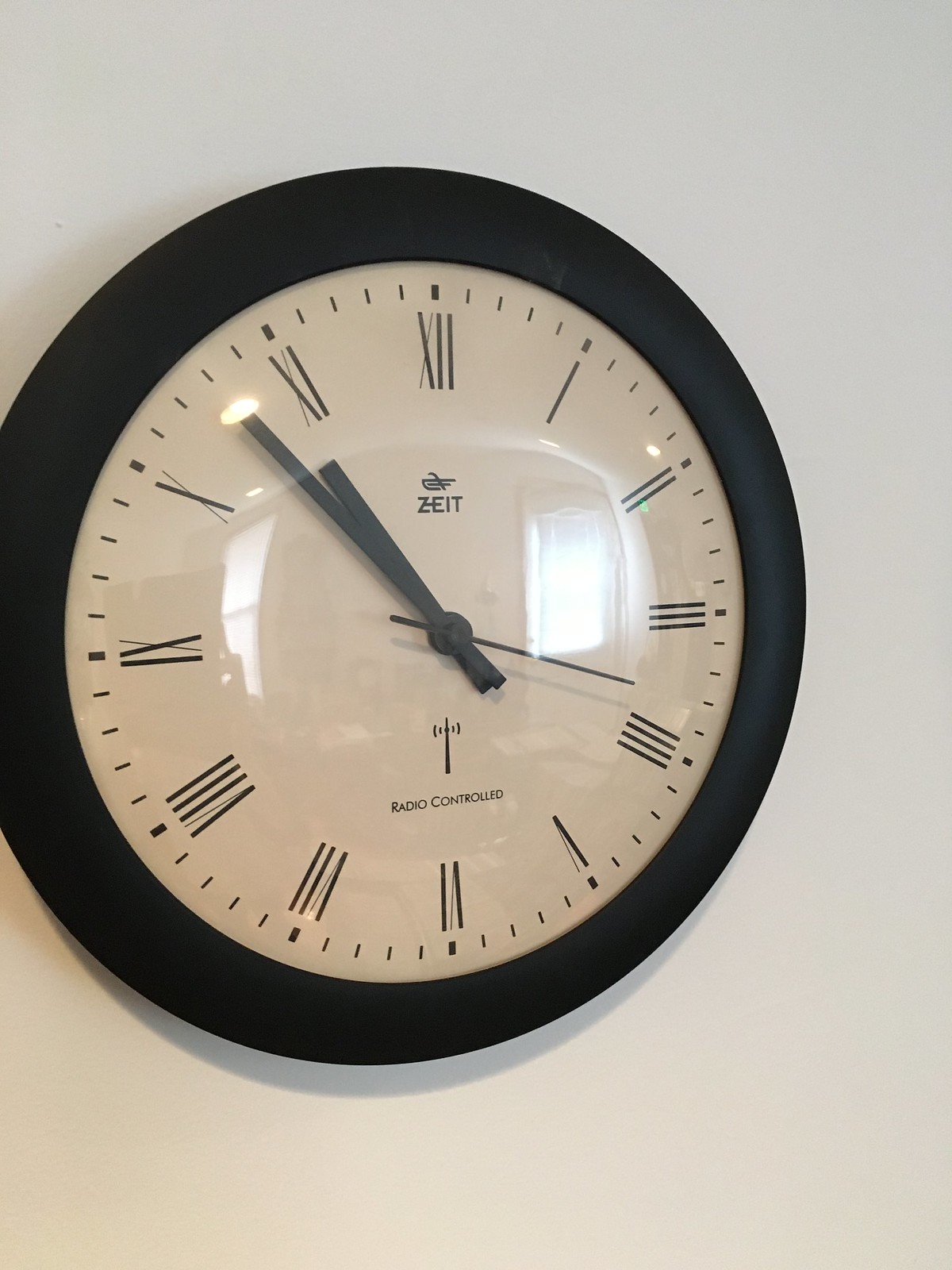The image features a wall-mounted clock set against a light gray, almost white background. The clock's face is a white, slightly pinkish-tan color and is encased by a thick black ring, potentially made of plastic or metal. The clock displays time with Roman numerals, complemented by thick dots marking the hours and thinner lines denoting the minutes. The clock's hands are black rectangles, with the shorter, thicker hour hand, longer minute hand, and a thin, skinnier second hand. The current time shown is approximately 10:54, with the second hand situated between the Roman numerals III and IV. Central to the design is the brand "ZEIT," prominently featured below the 12 o'clock mark, accompanied by a distinct black logo resembling a horizontal and vertical slash. Below the hands, another symbol resembling an antenna signifies the clock's radio-controlled feature, clearly labeled "Radio Controlled" beneath it.